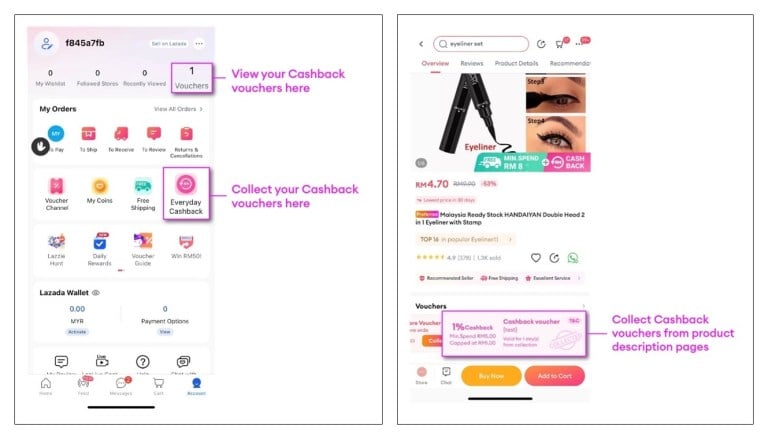The image features two vertically-aligned rectangular sections side by side. The left rectangle contains a user interface with several icons and text elements, though the resolution is low. 

- At the top, there's a circle with a person icon inside it. Below that, a sequence of alphanumeric characters reads "1-8-4-5-A-7-F-B" in black.
- Following this, there are sections labeled "My Wishlist," "Featured Stores," and "Recently Viewed," each accompanied by a zero.
- Further down, there's a section titled "Vouchers," highlighted in a purple box. Inside this box, it says, "View your cashback vouchers here."
- Below this, an "Everyday Cashback" icon is enclosed in another purple square, alongside text indicating, "Collect your cashback vouchers here."

To the right, in the second rectangle:
- There's a section bordered in purple labeled "1% cashback," which mentions a minimum spend, though the exact details are indistinct due to poor image resolution.
- Additionally, there appears to be a limit or cap described as "RM," but the specific figure is unreadable.
- A note on the side states, "Collect cashback vouchers from product description pages."

Despite the poor resolution, the image primarily seems to revolve around a user interface focused on cashback vouchers and featured shopping options.